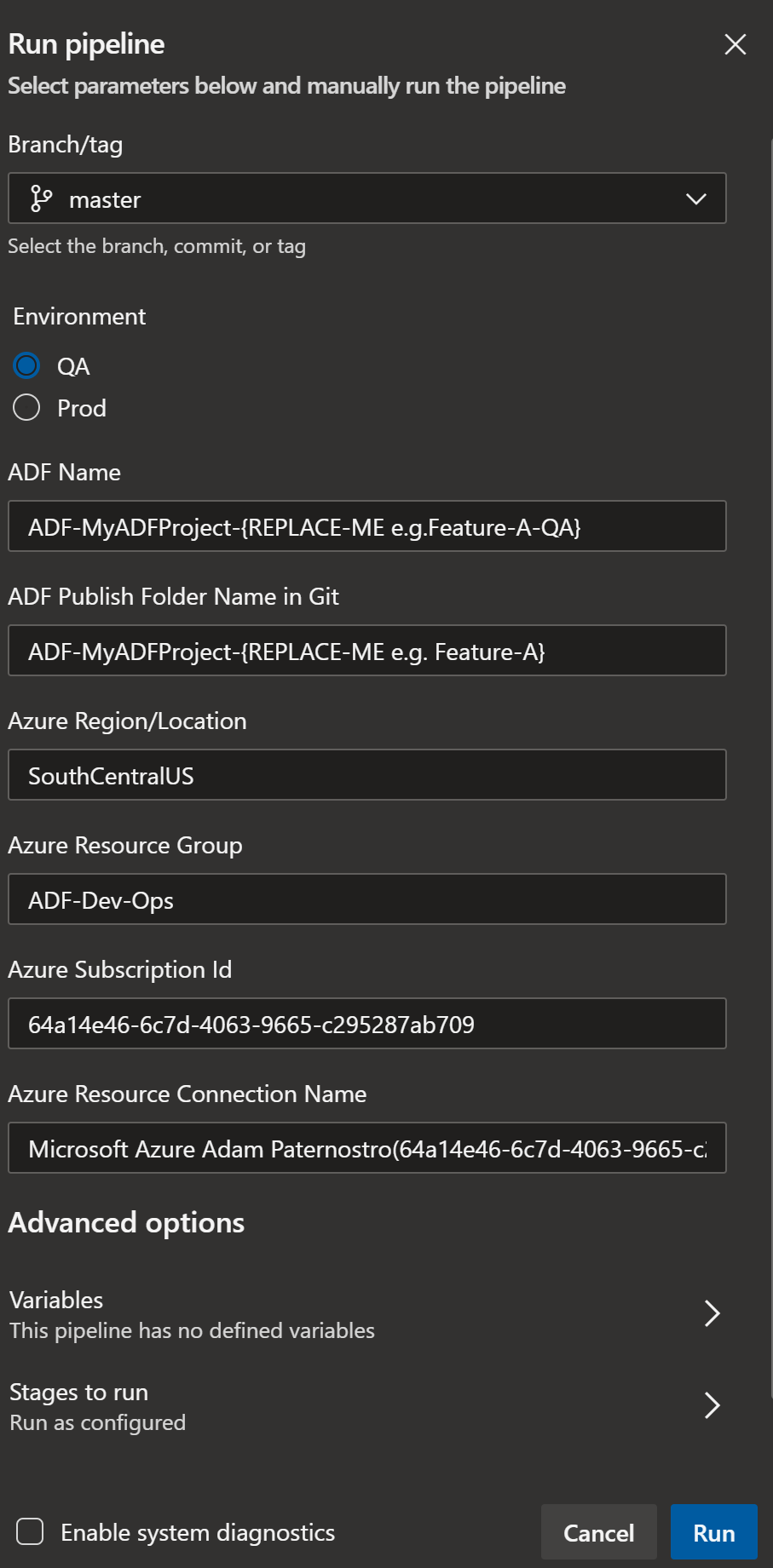The image depicts a user interface for running a pipeline within a software development environment. The background of the page is black, adorned with multiple input boxes and selection options designed to configure and execute the pipeline. The most prominent section invites the user to "Run Pipeline," followed by a prompt to "Select parameters below and manually run the pipeline."

The first input field is labeled "Branch / Tag," accompanied by a dropdown menu from which the user can select a branch, commit, or tag. In this instance, the selected option is "master." 

Next, there's an "Environment" section offering checkboxes labeled "QA" and "prod," with "QA" currently selected.

Following that is the "ADF Name" field, where the user has entered "ADF-my ADF project (replace-me e.g. feature a QA)."

Below this is the "ADF Publish Folder Name in Git" field, populated with "ADF-my ADF project-replace me e.g. feature A."

Further down, the "Azure Region / Location" is specified as "South Central U.S."

The "Azure Resource Group" is listed as "ADF-dev-ops."

The "Azure Subscription ID" is inputted as "64A14E46-6C70-4063-9665-C295287AB709."

The "Azure Connection Name" displays "Microsoft Azure Atom Paternstro."

Towards the bottom of the interface, the user has options for "Advanced Options," "Variables," "Stages to Run," and an option to "Enable System Diagnostics."

Finally, two buttons are available for user interaction: "Cancel" and "Run."